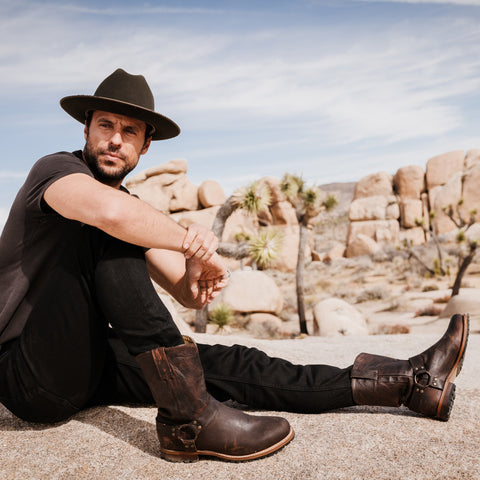In a sunlit desert landscape, a man in his 30s to 40s is seated on a gray rock with a relaxed yet contemplative posture. He's dressed in a black cowboy hat with a light-colored band, a black t-shirt, black jeans, and modern brown leather boots with circular buckles on the sides. His right leg is bent at the knee, while his left leg extends forward, and he rests his right elbow on his knee with his left hand clasping his right wrist. The man, bearded and inquisitive, gazes off to the left, casting shadows in the bright sunlight. Behind him, the scene is defined by rugged brown boulders, green desert plants including cacti—identified possibly as Joshua trees—and a pale blue sky adorned with wispy clouds, suggesting he might be in a southwestern desert environment, like Palm Springs. The photograph's context is unclear, leaving it open to interpretation whether it is a candid moment, a modeling shoot, or a self-portrait using a tripod.